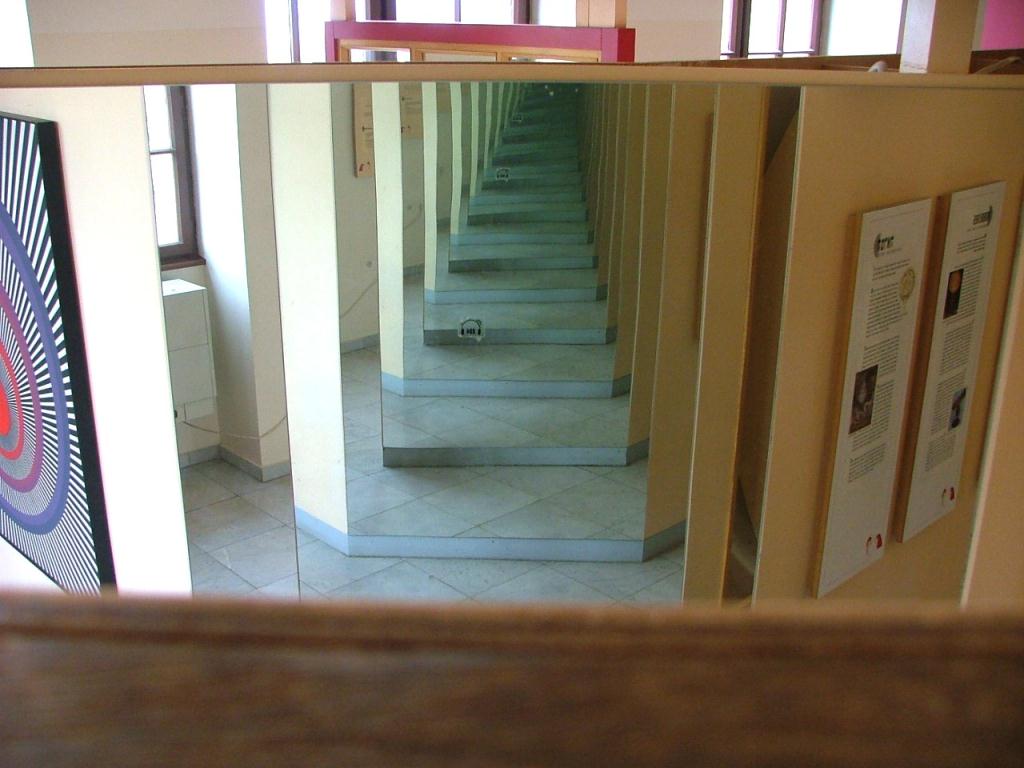The image depicts a clever optical illusion created by two mirrors facing each other, generating an infinite recursive reflection. The primary feature in the center appears to be a staircase illusion formed by the repeating mirrors, which reflect the diamond-patterned gray tile floor. This continuous reflection creates a visual effect of ascending steps into the background. On the left-hand side of the image, there's an intriguing piece of art characterized by diagonal lines and a central spiral, producing a hypnotic optical illusion. To the right of the mirrored area, there are wall plaques densely packed with text and small, indistinguishable images, suggesting a public setting. The image's angle is tilted slightly downward, intentionally avoiding the camera's reflection, further enhancing the illusion of an endless tunnel.